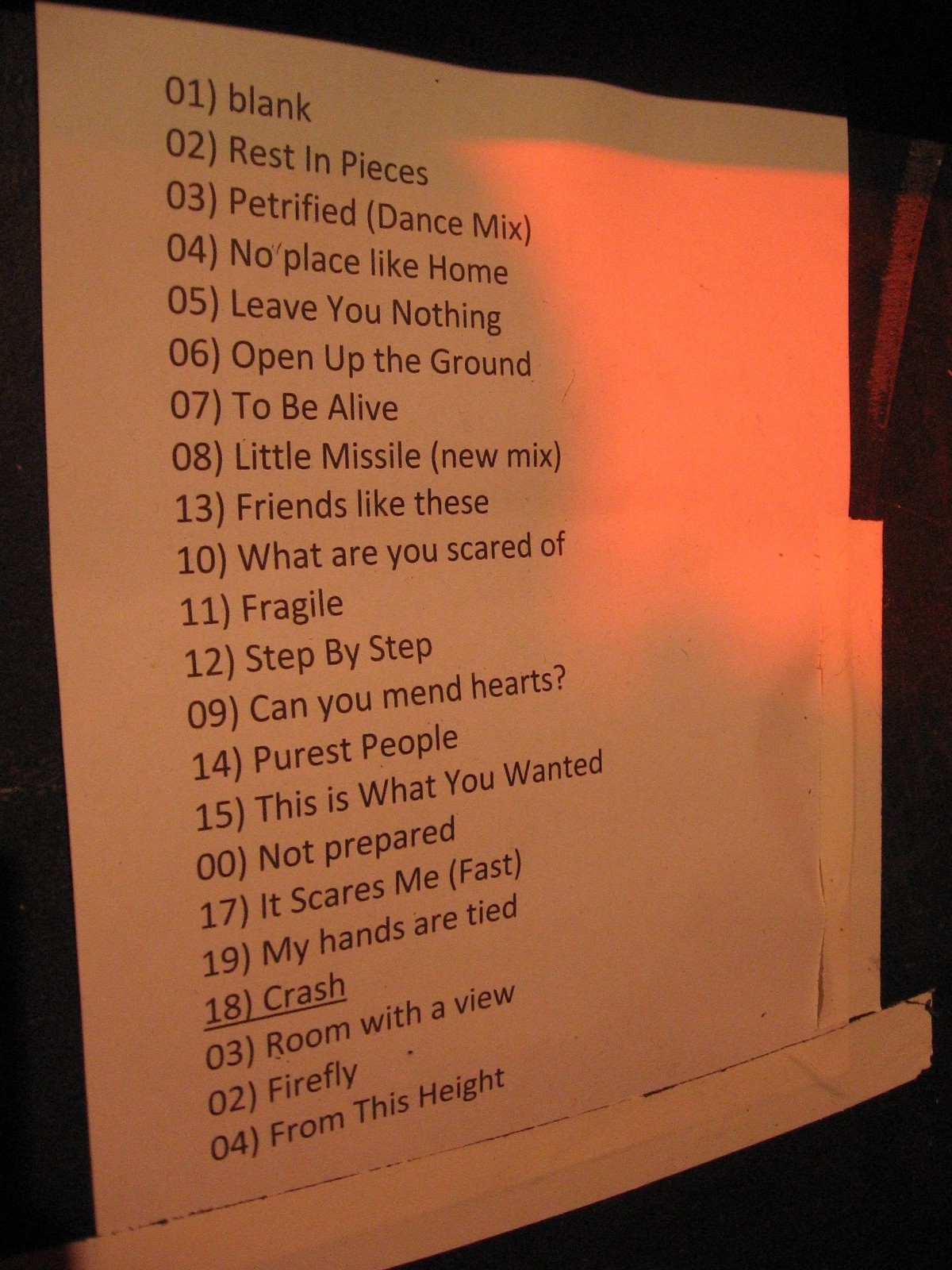This detailed photograph features a white piece of poster board, presumably affixed to a wall with white duct tape visible near its bottom edge and side, suggesting it is otherwise unsupported and dangling slightly. The poster itself is situated in a dimly lit room, with a shadowed left side and a red-filtered light striking it from the right. The poster lists what appears to be a series of song titles, printed in black text on a white background and includes numbers that are not in a sequential order. The list includes: 

- 01 (Blank)
- 02 (Rest in Pieces)
- 03 (Petrified Dance Mix)
- 04 (No Place Like Home)
- 05 (Leave You Nothing)
- 06 (Open Up the Ground)
- 07 (To Be Alive)
- 08 (Little Missile New Mix)
- 13 (Friends like These)
- 10 (What Are You Scared Of?)
- 11 (Fragile)
- 12 (Step-by-Step) 
- 09 (Can You Mend Hearts?)
- 14 (Purest People)
- 15 (This Is What You Wanted)
- 00 (Not Prepared)
- 17 (It Scares Me Fast)
- 19 (My Hands Are Tied)
- 18 (Crash), with ‘Crash’ being underlined
- 03 (Room with a View)
- 02 (Firefly)
- 04 (From This Height)

There are no images or graphics on the poster; it contains solely text, each title formatted with specific capitalization and punctuation styles. At the bottom of the image, a white windowsill is discernible, adding further context to the setting of this peculiar and somewhat cryptic display.